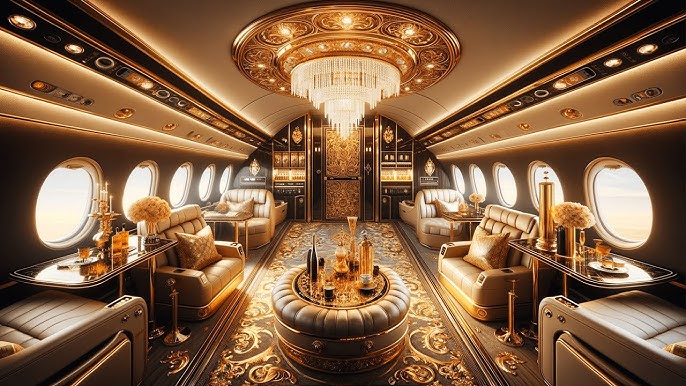This image depicts the luxurious interior of a private jet, characterized by an opulent golden color scheme. Dominating the ceiling is an elegant chandelier adorned with white or crystal beads and surrounded by golden lights, casting a warm glow over the room. The ceiling itself features a light brown hue with dark strips running along the edges.

The seating arrangement includes six plush, leather light brown chairs—three on each side—each positioned beside glass tables displaying an assortment of alcoholic drinks and floral arrangements. In the center of the cabin, a circular table holds clear bottles filled with golden liquid and glasses, accentuating the lavish atmosphere. The floor boasts intricate golden designs set against a brown backdrop, enhancing the cabin's grandeur.

Detailing extends to black and gold elements spread throughout, including gold canisters, candlesticks, and pillows with golden patterns. The door leading to the pilots' area is also adorned in gold and dark accents, maintaining the consistent theme of luxury. The view through the windows shows the sky, confirming that this extravagant setting is, without a doubt, inside a first-class private jet.